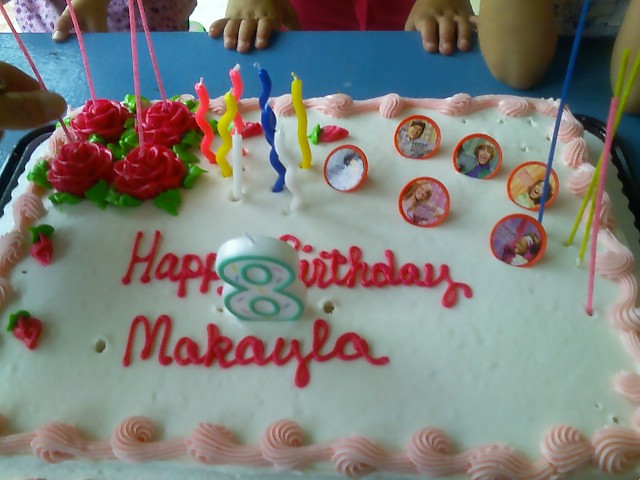This close-up color photograph showcases a beautifully decorated rectangular birthday cake set against a blue table, with a few brown-skinned children's fingers gripping the table's edge. The cake is adorned with smooth white frosting and intricate pink swirls around its edges. In the upper left corner, there are four realistic red frosting roses with light green leaves, each rose featuring a pink sparkler. Scattered across the cake are diverse candles, some twirly in blue, pinkish-red, yellow, and white hues. Sitting prominently at the center is a large plastic number "8" candle, symbolizing the celebrant’s age. Written in bright red icing at the center of the cake is the celebratory message, "Happy Birthday Makayla." The name is misspelled as "Michaela" in one account, but the correct spelling, "Makayla," is clear from the frosting. Additionally, there are small circular decorations that appear to have tiny photographs on the right side of the cake. The scene captures the festive atmosphere of a child’s 8th birthday celebration.